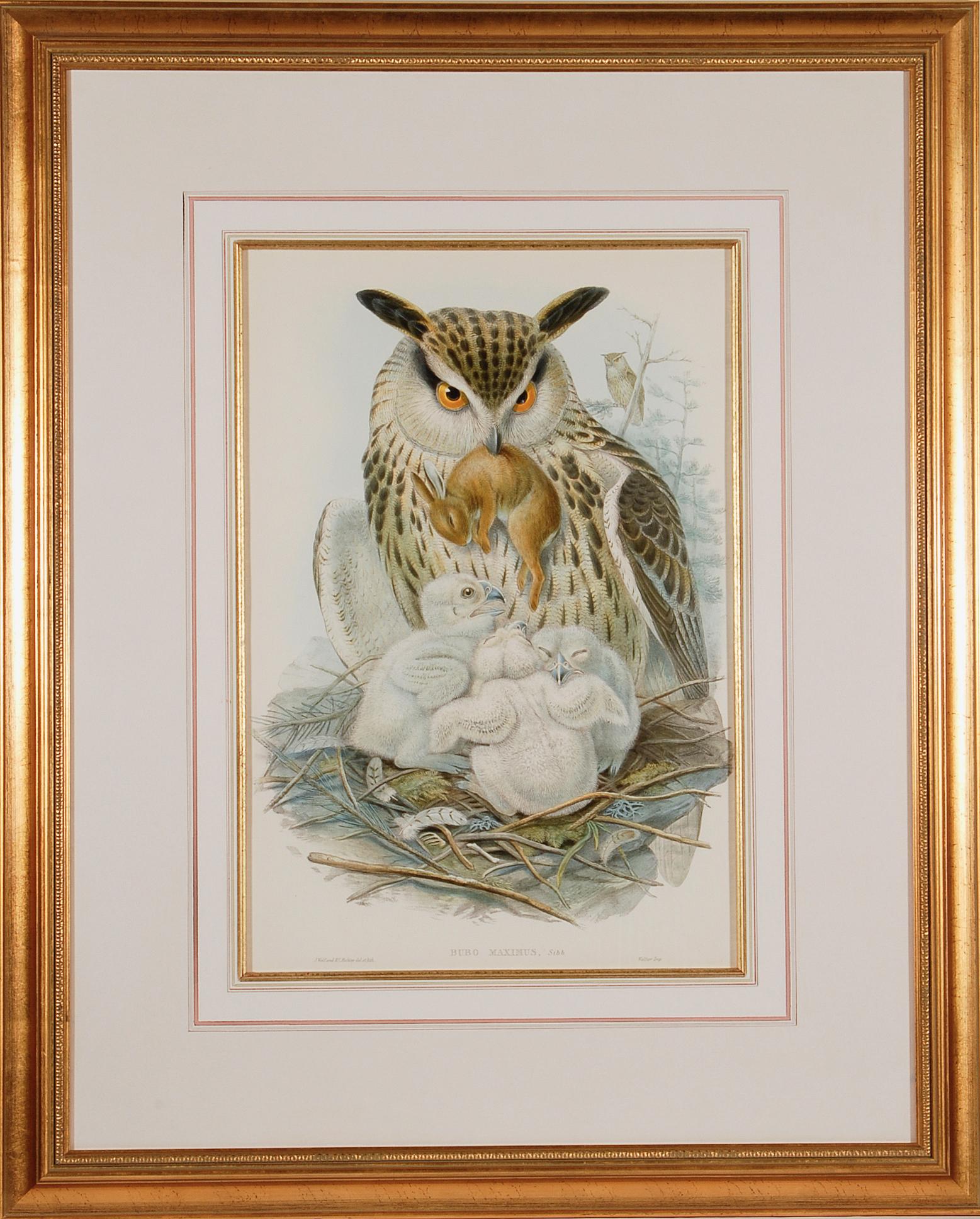This detailed artwork, elegantly framed in a gold rectangular border with a layered white mat and inner gold and white accents, depicts a captivating scene of nature. Central to the image is a light brown and dark-spotted owl with prominent golden eyes and delicate black ear tufts, perched against a soft cream background. The owl, facing slightly right with its head turned down, grasps a small, lifeless brown rabbit in its gray beak, seemingly preparing to feed its three owlets nestled below. The baby owls, still covered in fluffy down feathers, huddle together in the nest with one looking up expectantly, another with eyes closed, and the third glancing to the side. In the serene background, muted trees provide a natural sanctuary where another owl perches on a branch. This striking depiction embodies the raw, nurturing essence of wildlife through its meticulous details and dynamic composition.